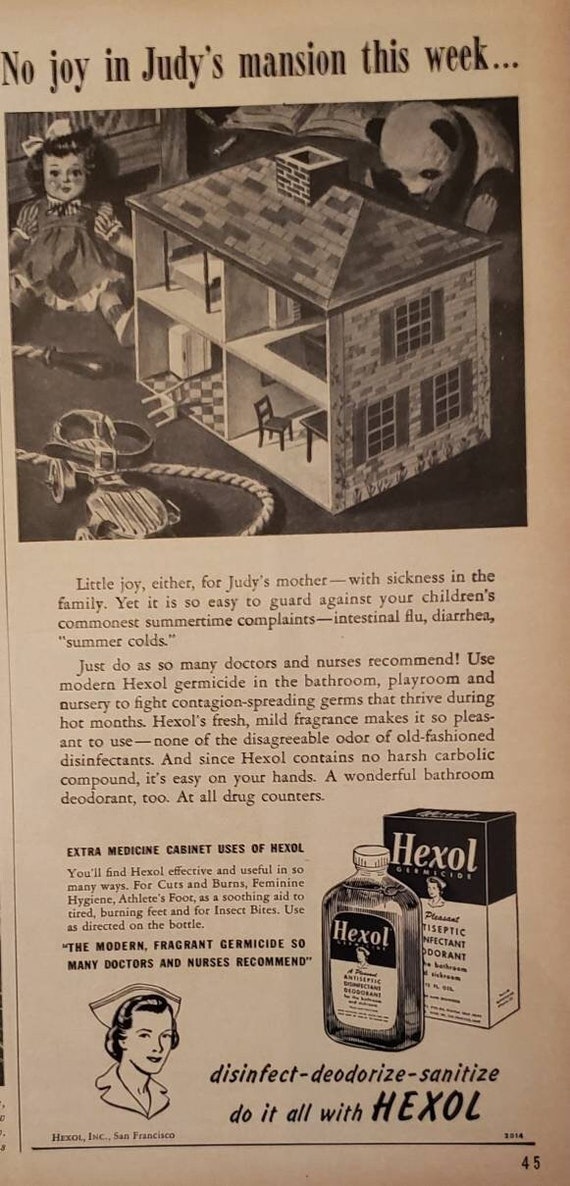This black-and-white vintage advertisement, which likely appeared in a magazine or newspaper, showcases an old-fashioned yet well-preserved look. At the top, the title reads "No Joy in Judy's Mansion this Week," drawing attention to a nostalgic scene featuring a dollhouse and a doll. Below the image, the first paragraph highlights a common concern from the time: "Little Joy, either for Judy's mother, the sickness in the family, yet it is so easy to guard against your child's commonest summertime complaints, intestinal flu, diarrhea, summer colds."

In the next section, the advertisement emphasizes various applications of Hexol, referring to it as "Extra Medicine Cabinet Uses of Hexol." It goes on to describe Hexol as "The Modern Fragrant Germicide So Many Doctors and Nurses Recommend." To the right of this text, an illustration prominently displays a box and a bottle of Hexol, with the product's name spelled out clearly.

In the bottom left corner, there is a partial image of a nurse's head, neck, and collar. Beneath the bottle on the right, the caption encourages consumers to "Disinfect, Deodorize, Sanitize, Do It All with Hexol." This captivating ad was featured on page 45 of the publication, making a compelling case for Hexol as a trusted household germicide.